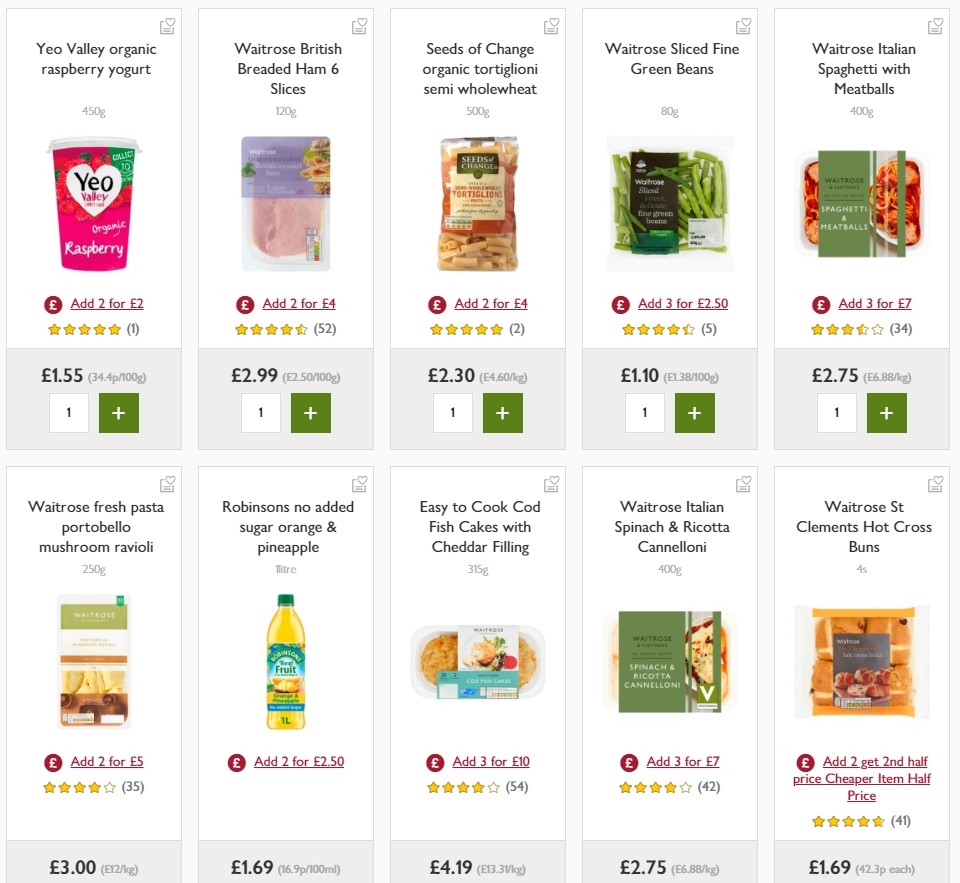The image features a variety of products along with their prices. At the top of the image is E.O. Valley Organic Raspberry Yogurt, priced at €1.55. Next is White Toast British Bread and Ham, containing 6 slices, available for €2.99. Adjacent to it, there is Seeds of Change Organic Tortellini made with Semi-Whole Wheat, costing €2.30. The next item listed is White Toast Sliced Fine Green Beans, priced at €1.10. 

Below that, there is White Toast Italian Spaghetti with Meatballs, available for €2.75. Another pasta option shown is White Toast Fresh Pasta Portobello Mushroom Ravioli, which costs €3.00. Additionally, there is Robinson's No Added Sugar Orange and Pineapple juice, priced at €1.69.

Next on the list are Easy-to-Cook Codfish Cakes with Cheddar Filling, available for €4.19. This is followed by White Toast Italian Spinach and Ricotta Cannoli, priced at €2.75. Lastly, there are White Toast St. Clement's Hot Cross Buns, which cost €1.69 each.

The image also highlights promotions such as "Add 3 for €7," "Add 3 for €2.50," and "Add 3 for €10."